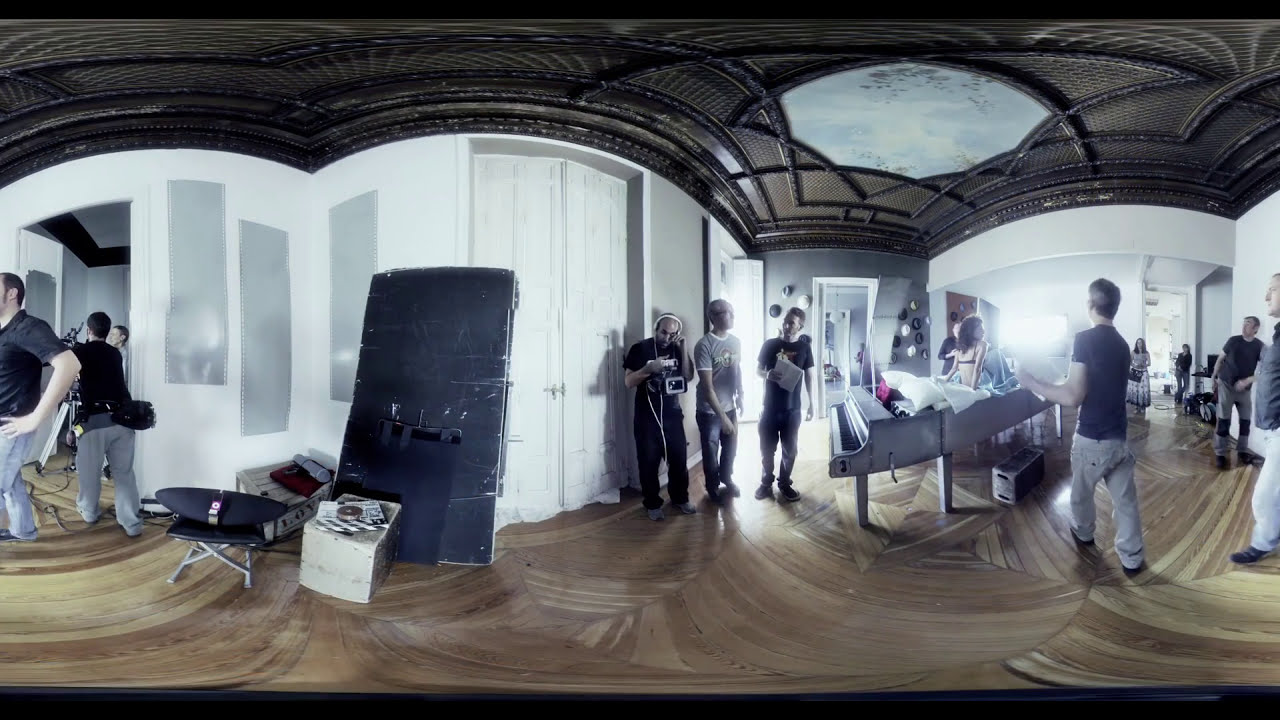The image is a 360-degree view of a spacious room with a unique combination of elements suggesting a filming scene, possibly for a music video. The room features white walls with three mirrors mounted on the left side and intricate wooden paneled flooring. The ceiling is constructed of metal and has a woven brown material, with a circular skylight at the center. A thin black line runs horizontally along the top and bottom of the image.

At the heart of the room are large double white doors, closed, with three men standing in front of them. One of the men is notable for wearing white headphones and dressed in black, carrying a camera mounted on his chest.

Positioned to the right of these men is a piano, with another piano directly opposite it. A woman, dressed in a black bra and wrapped in a blue blanket with white pillows behind her, is sitting upright on this piano. The piano is a wind-up type, with the keyboard section behind her. Near her, a prominent light is set up, indicating a filming setup, with cords scattered on the floor nearby. 

To the left, equipment and a wooden crate marked with the word "Love" can be seen. Additionally, a guy holding papers, wearing a gray shirt, is seen discussing with another man. The room is filled with various people, some milling about and others watching the scene unfold, adding to the dynamic atmosphere of this busy, well-lit space.